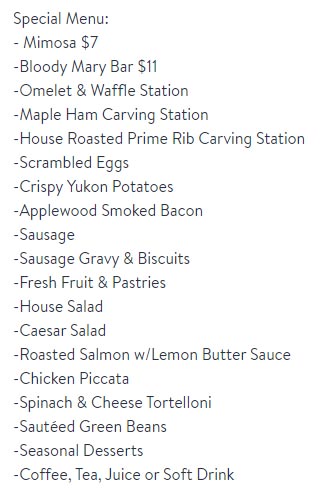A clean and detailed caption for the image could be:

"A screenshot featuring a simple, white-background catering menu titled 'Special Menu:'. The text is black and each menu item is listed with a hyphen. The first two items are Mimosa - $7 and Bloody Mary - $11, which include prices. The following items do not have prices listed and include: Omelet and Waffle Station, Maple Ham Carving Station, House Roasted Prime Rib Carving Station, Scrambled Eggs, Crispy Yukon Potatoes, Applewood Smoked Bacon, Sausage, Gravy and Biscuits, Fresh Fruit and Pastries, House Salad, Caesar Salad, Roasted Salmon with Lemon Butter Sauce, Chicken Piccata, Spinach and Cheese Tortellini, Sautéed Green Beans, assorted Desserts, Coffee, Tea, Juice, and Soft Drinks."